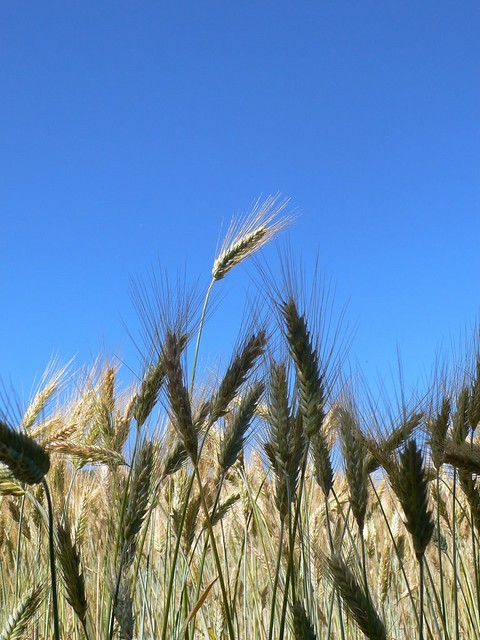The image features a close-up view of a field of wheat, with hundreds of light golden-brown stalks rising against a clear, bright blue sky. The camera angle shoots upward from within the field, accentuating the wispy and somewhat shadowed heads of wheat due to the backlighting. Dominating the scene, one prominent stalk of wheat stands out, extending above and catching the sunlight. The overall composition captures the serene simplicity of the wheat field and the vast openness of the sky, with no other elements present in the frame.